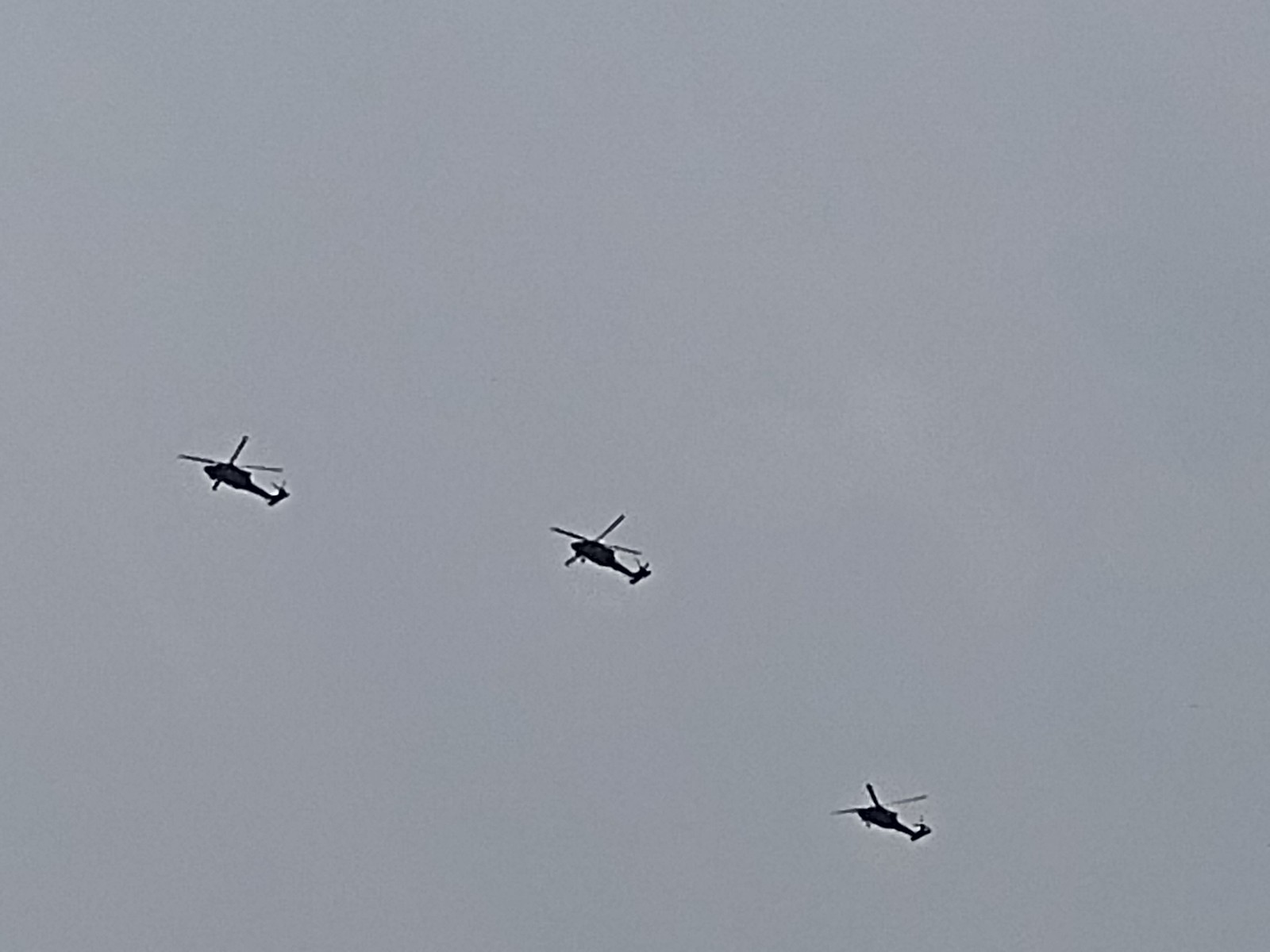The photograph captures an outdoor daytime scene with a grayish-blue sky filling the entire image, indicating that the photographer directed the camera upwards. The picture is in landscape orientation and features three four-bladed helicopters flying in formation across the sky, silhouetted against the backdrop. Despite the grainy texture of the image, the helicopters are in relatively sharp focus compared to the vague background. Positioned at varying heights, one helicopter is about halfway up the left side, another is centrally located, slightly higher, and the third is near the bottom right. They all appear to be modern military helicopters, but the distance makes it impossible to discern further details such as their color or national origin. The sky is uniformly clear, devoid of clouds, text, or any other foreground elements, emphasizing the stark formation of the helicopters against the expansive sky.